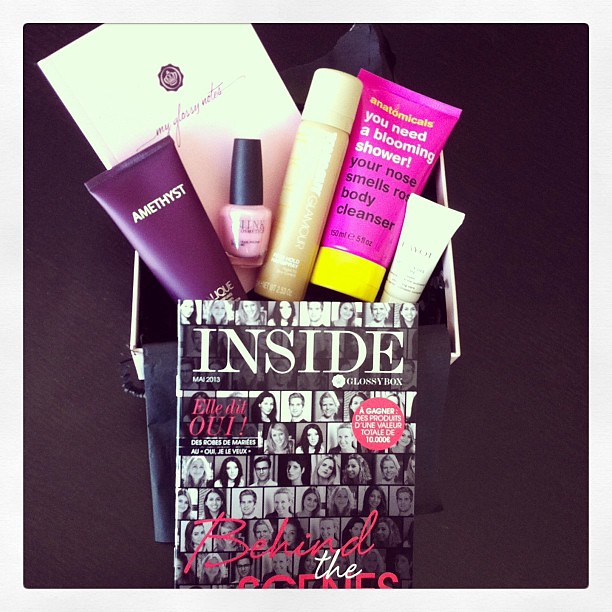The image features a dark backdrop highlighting an arrangement of beauty and skincare products with a magazine cover prominently positioned. The magazine, titled "Inside," is displayed in the lower left center of the image. It showcases a monochrome layout filled with rows of headshots underneath the title. Resting horizontally behind the magazine is a white box with a black interior and possibly a brown cloth lining. 

On top of the box and around it are five distinct beauty products and a card labeled "My Classy Notes." Among these products, a purple tube reading "Amethyst" in white letters stands out prominently. Additionally, there is an eyeliner with a pink bottom and a black cap, a gold/yellow tube, and a neon/hot pink bottle labeled "anatomicals, you need a blooming shower, your nose smells rose body cleanser." A smaller white tube is included in the assortment, enhancing the diversity of products featured. The vibrant colors and elegant packaging set a striking contrast against the magazine and its more subdued tones.